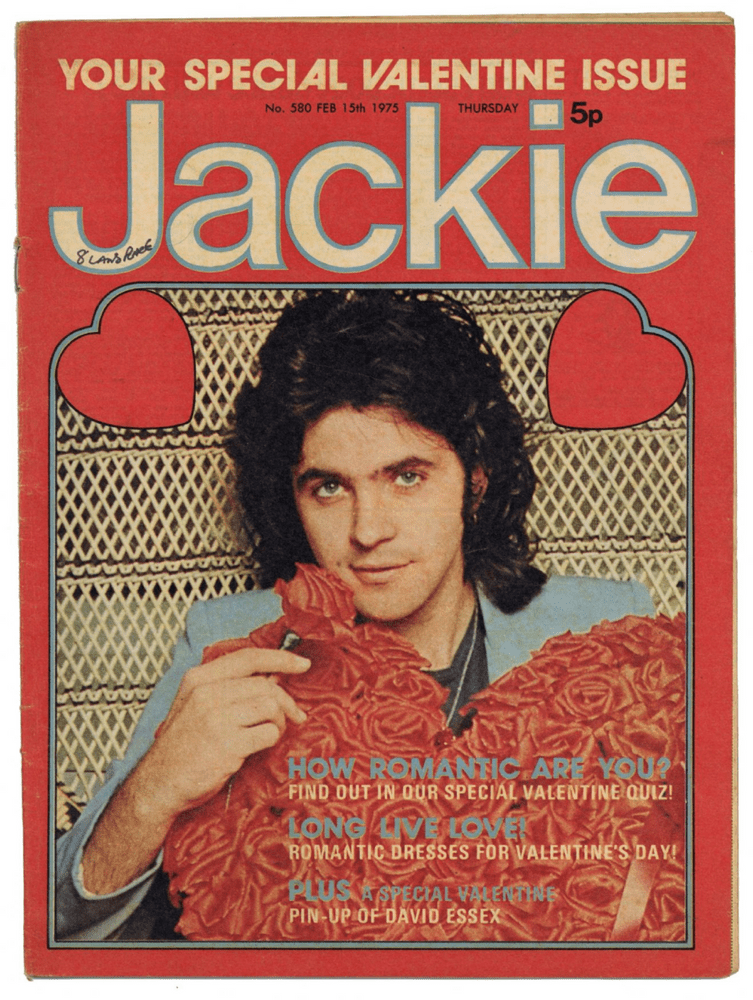The vintage magazine cover, predominantly red, features the title "Jackie" in large white text with a light blue outline, along with the heading "Your Special Valentine Issue" in smaller white text. Priced at 5 pence and published in the United Kingdom, this particular edition is Issue No. 580, dated Thursday, February 15th, 1975. Dominating the cover is an image of a man with brown mullet-style hair and blue eyes, dressed in a light blue suit jacket with notably short sleeves. He is depicted holding a bunch of red roses shaped like a heart, surrounded by two hearts around his head. Additional cover lines include enticing phrases such as "How romantic are you", "Long Live Love", and more, underscoring the Valentine's Day theme.